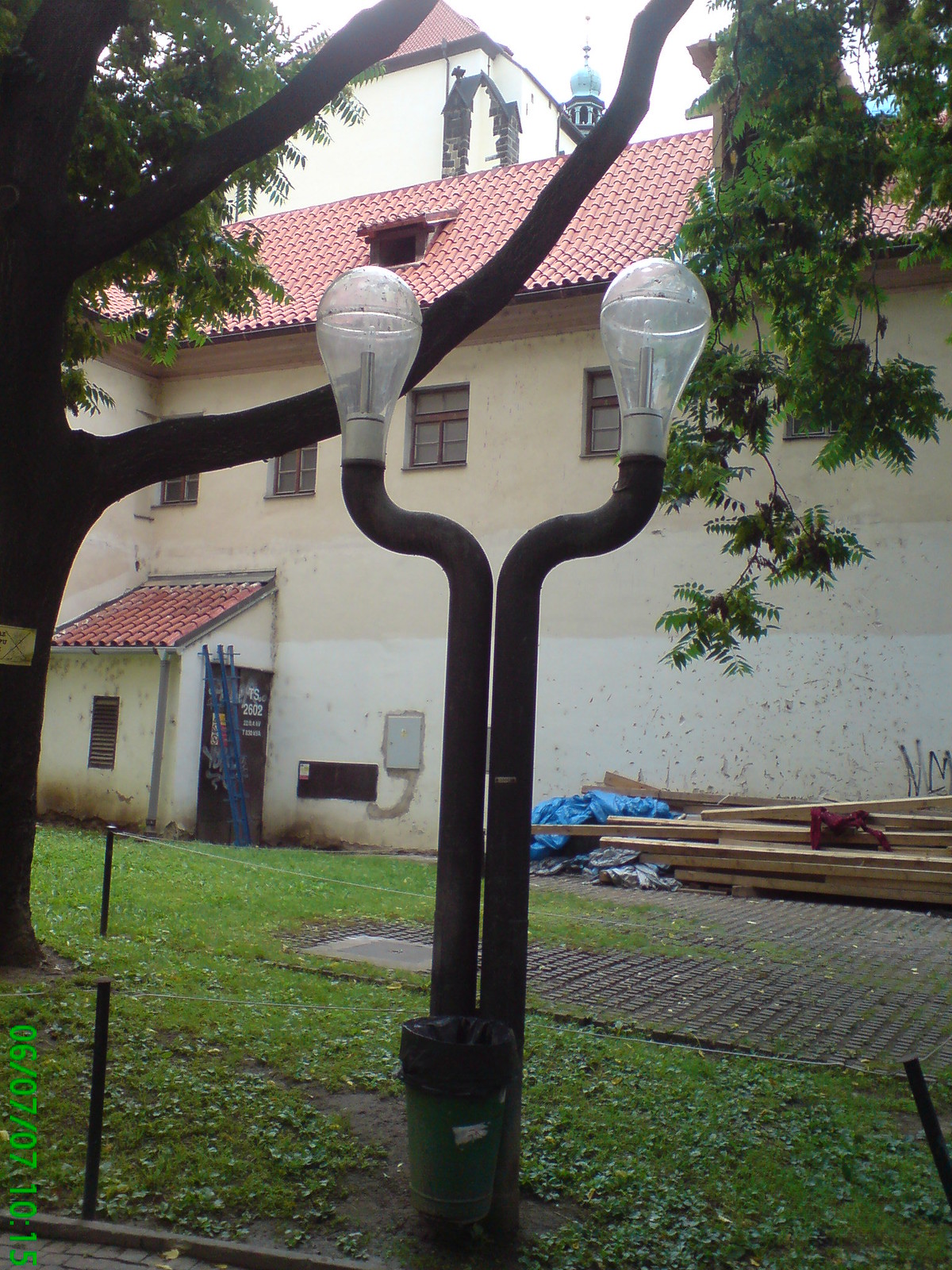In this photograph taken on June 7, 2007, at 10:15 AM, we see a pair of distinctive street lamps situated in an outdoor setting. The lamps, crafted from black metal, stand very close together, with their poles elegantly curling outward at the top to form a gentle U-shape. Each pole supports a large bulb encased in a hazy, possibly plastic, cover, revealing a shiny metallic cylinder and a small light bulb inside. At the base of the poles, there's a small green trash can, fitted with a black bag.

The scene features a building in the background, taking up much of the space. The structure, a likely church with a steeple bearing a crucifix, has a two-toned facade—its bottom half a whitish color and its top half a beige. The building also sports a striking bright red roof and has several small, square windows near the top. A large tree is positioned on the left side of the image, casting a shadow on the lamp poles. Additional details include a stack of lumber and some tarps marked "NM" against the wall on the building's right side. Sparse green grass covers the ground, giving the entire image a slightly untidy look, accented by a muddy patch where the lamps stand. The caption "0607071015" appears at the bottom left corner of the photo.